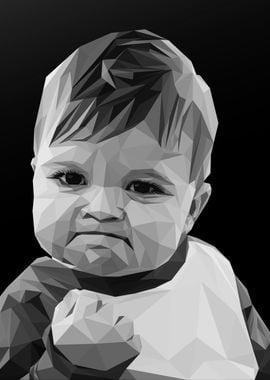This detailed black-and-white image features the well-known "Success Kid" meme, which depicts a young boy, about 2 or 3 years old, with short dark hair, standing at the center of the frame. The background is entirely black, emphasizing the child's intense expression. The boy's mouth is set in a downturn, and his eyes carry a menacing, determined look. He is holding his right fist up near his face in a triumphant gesture. The image has been artistically modified to appear as if composed of numerous triangles, giving it a geometric, almost three-dimensional quality. The boy's white shirt contrasts starkly against the dark background, and the texture of the image shows varying shades of black, gray, and white, creating a metal-like effect. The left ear is barely visible, further adding to the image's unique, fragmented appearance.